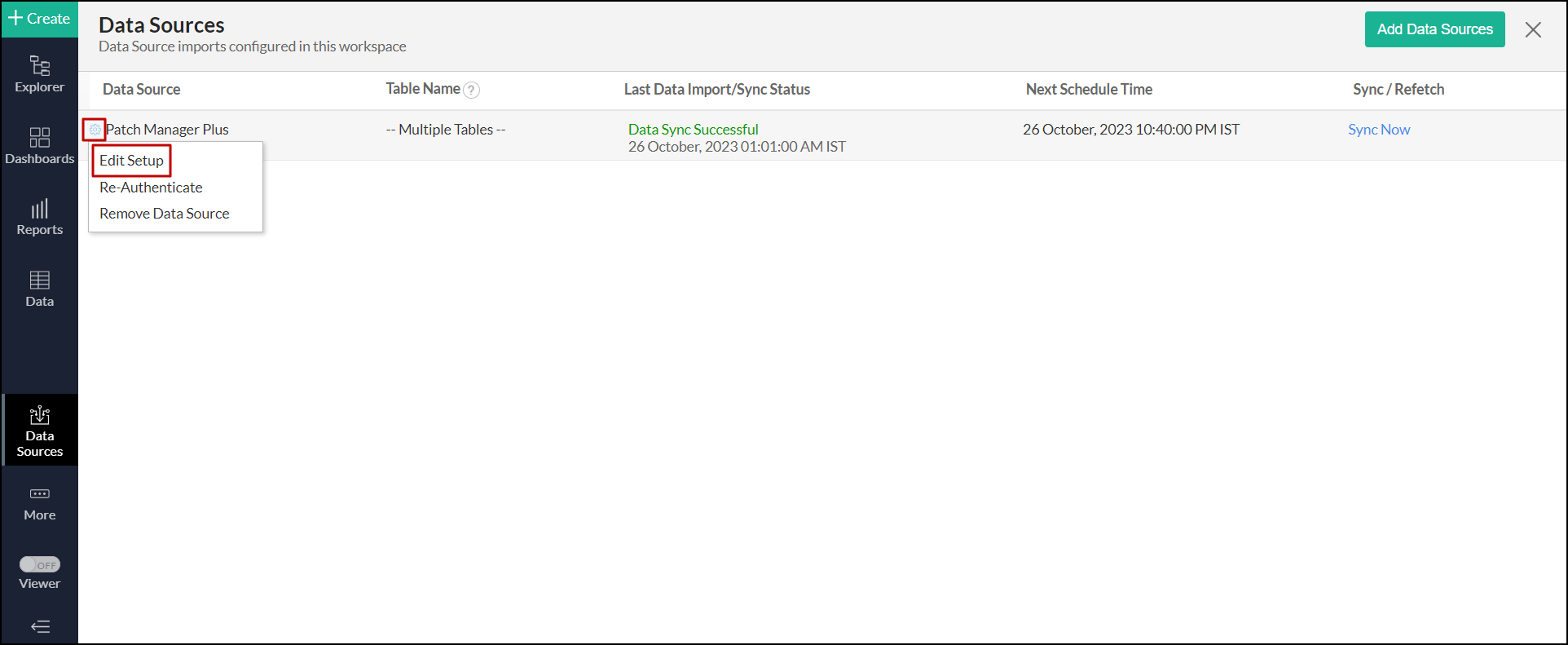The image features a detailed interface for managing data sources. On the left-hand side, there is a vertical navigation sidebar. At the very top of this sidebar, there is a "Create" option accompanied by a small plus (+) button. Below the "Create" button, the sidebar lists several options: "Explorer," "Dashboards," "Reports," "Data," "Data Sources," "More," and "Viewer." The "Data Sources" option is slightly highlighted, indicating it is the currently selected section.

The main section of the page prominently displays the heading "Data Sources" at the top, followed by a subheading that reads, "Data source imports configured in this workspace." On the far right of this main section, there is a prominent green button with white text labeled "Add Data Sources."

Below the subheading, there is a tabular list consisting of a single entry. The table is organized into five columns: 
1. Data Source
2. Table Name
3. Last Data Import/Sync Status
4. Next Schedule Time
5. Sync/Refetch

Each column provides specific information relevant to the data source management, and the solitary entry is displayed accordingly under these headers.